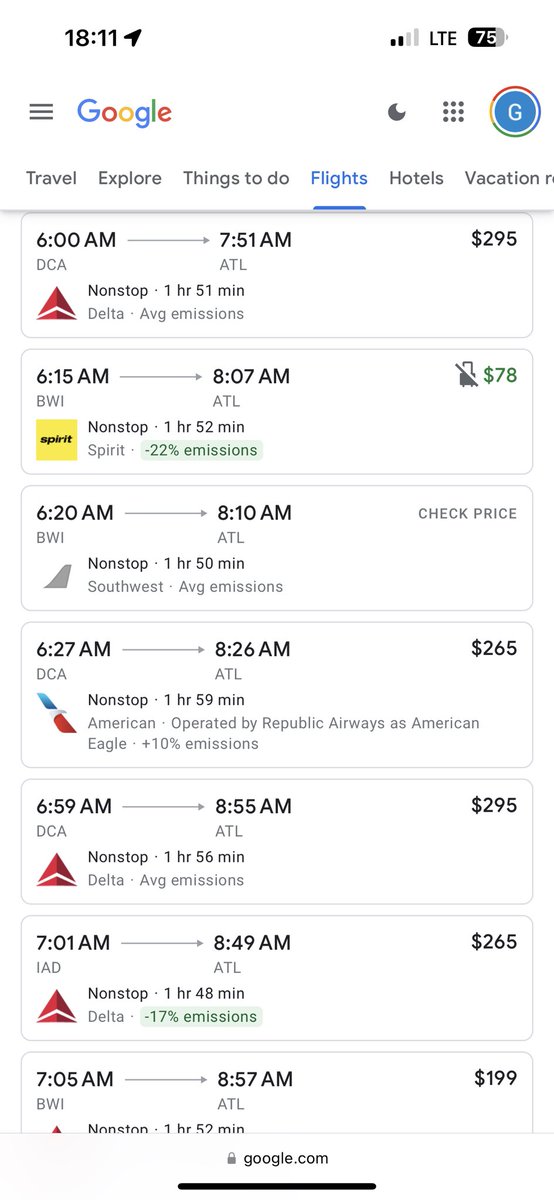The image depicts a cell phone screen displaying flight search results. The status bar at the top shows the time as 18:11 in the upper left corner, with cellular signal strength, LTE connectivity, and a battery icon at 75% in the upper right corner. Below the status bar, the Google logo is prominently displayed, followed by a navigation menu with options: Travel, Explore, Things to Do, Flights (highlighted), Hotels, and Vacation.

The first flight listed departs from DCA to ATL, scheduled from 6:00 a.m. to 7:51 a.m., priced at $295 for a nonstop, 1 hour and 51-minute flight with Delta, labeled as having average emissions. 

The second flight, highlighted, is from BWI to ATL, departing at 6:15 a.m. and arriving at 8:07 a.m., priced at $78. This nonstop flight with Spirit Airlines has a duration of 1 hour and 52 minutes and is noted for having 22% lower emissions.

A third option shows a flight from BWI to ATL, departing at 6:20 a.m. and arriving at 8:10 a.m., with a "Check Price" prompt. This nonstop flight is operated by Southwest and lasts 1 hour and 50 minutes with average emissions.

Multiple other flight options are listed, all heading to Atlanta (ATL) with departure times between 6:15 a.m. and 7:05 a.m., and arrival times between 8:07 a.m. and 8:57 a.m. Each flight varies in price, with costs displayed along the right side of the screen.